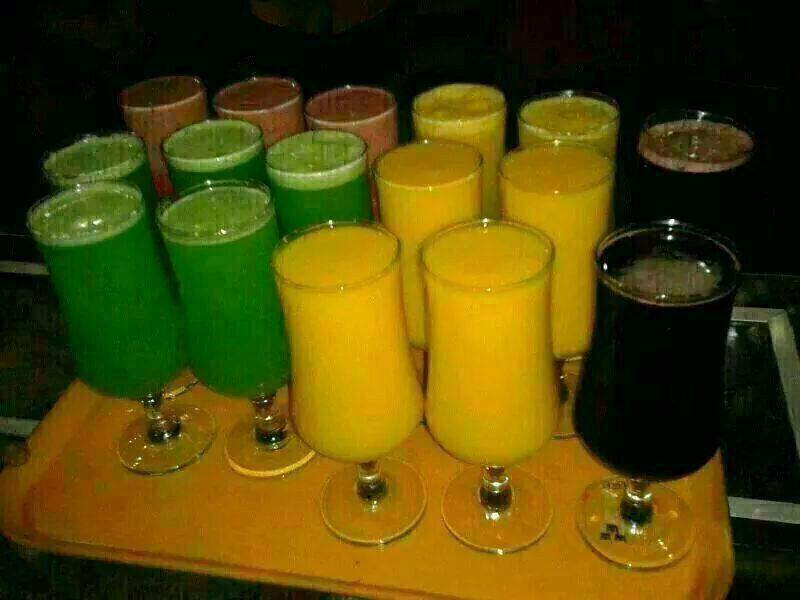The image shows a wooden serving tray placed on a table with a silver-edged outline, set against a dark, black background. Arranged on the tray are 16 vibrant drinks in tall, curvy, stemmed glasses. On the left side, there are five green drinks, likely smoothies or cocktails, followed by three reddish-orange beverages behind them. Positioned centrally are six yellow drinks, likely resembling mimosas or orange juice. On the far right, two dark brown or possibly cola drinks are noticeable. The overall scene suggests a festive setting, with the glasses uniformly styled, prepared to be served in a dimly lit environment.